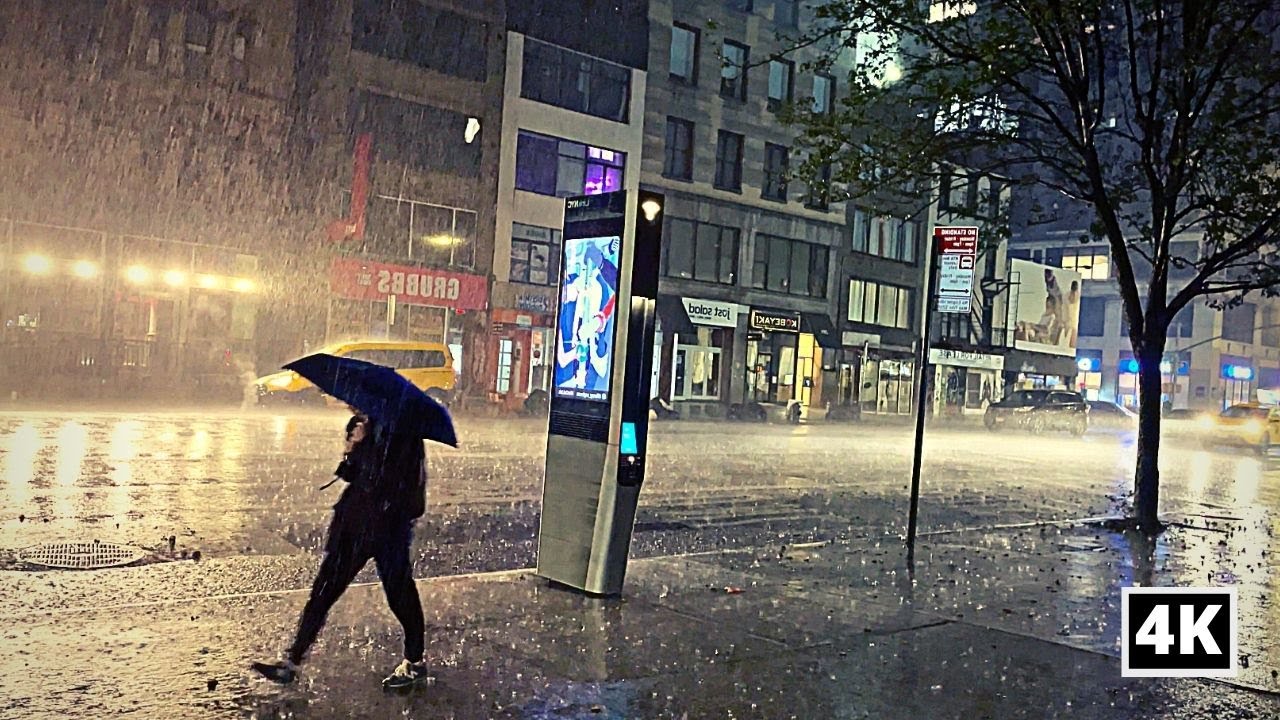In this vivid and sharp urban scene captured on a rainy day, an individual clad in dark clothing huddles under a dark umbrella as they walk on the rain-soaked sidewalk. Positioned in the bottom left of the image, the person is heading past a brightly lit, towering advertisement display, roughly 8 to 9 feet tall, which casts a glow over the wet pavement. In the far right corner of the photograph, the sharp quality of the image is endorsed by the "4K" label. The heavy downpour is almost palpable; each droplet is crisply defined, intensifying the dreary yet compelling atmosphere.

Surrounding the person are telltale signs of urban life: a single tree grows from the sidewalk's edge, next to a parking restriction sign, and multi-story buildings line the street. Across the street, a yellow taxi cab and several other cars with their headlights on can be seen amidst a backdrop of bustling storefronts, their signs slightly blurred or reversed, enhancing the sense of a living, breathing city. This clear, modern photograph captures a fleeting moment of solitude amidst the relentless pace of city life, where even in the rain, activity never stops.